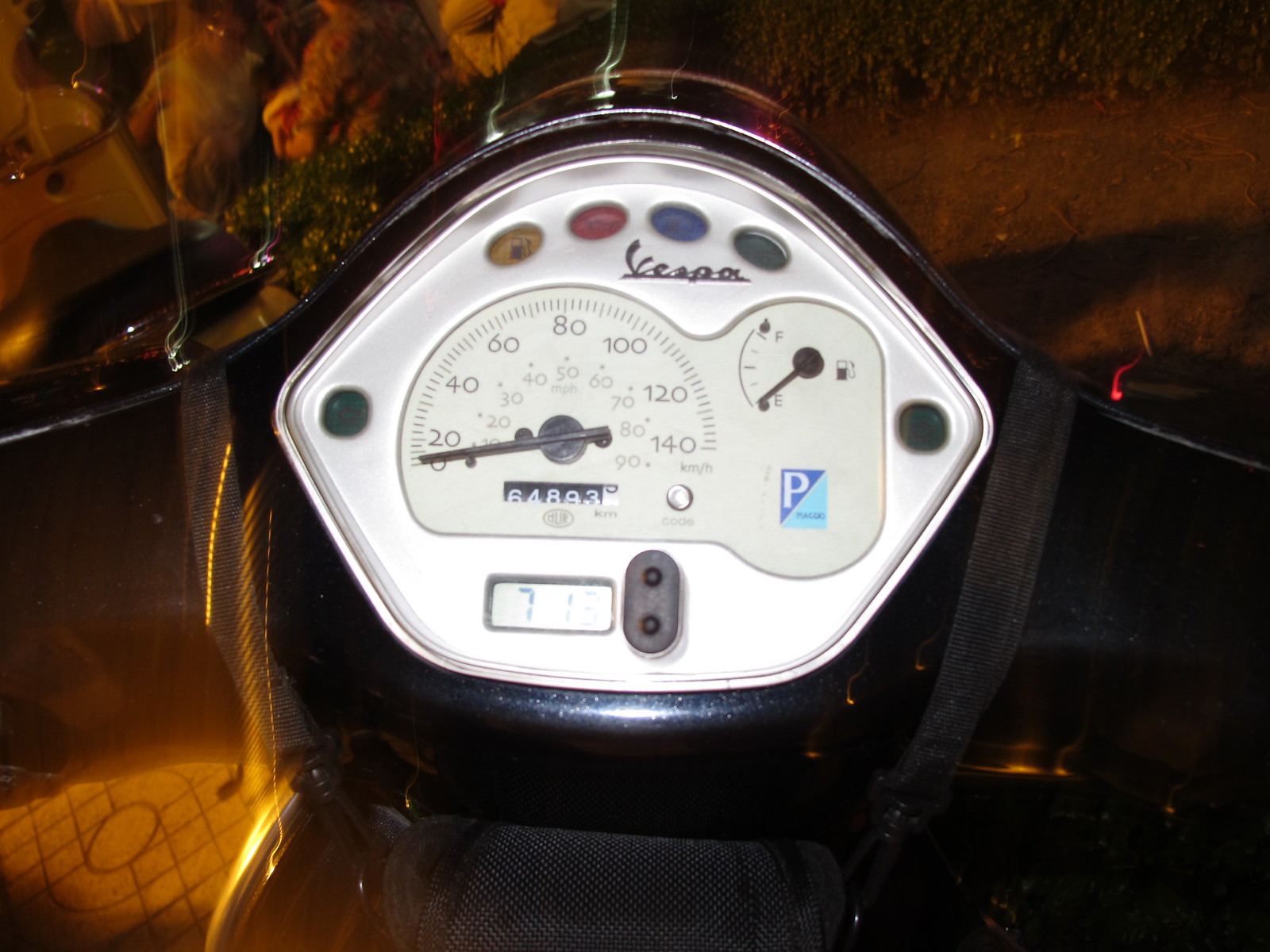This photograph captures the control board of a Vespa scooter, providing a glimpse into its intricate details. The image prominently features the handlebars and the upper section where the headlight is located, extending slightly towards the seat area. The Vespa appears to be parked outside under low lighting conditions, with the camera's flash giving a distinct illuminated effect. 

The surroundings reveal a piece of the sidewalk, part of a curb, green grass, and a few flowers, indicating a natural outdoor setting. The Vespa's screen is bright white, suggesting it is not turned on, as none of the indicator lights are lit. However, colorful lights on the control panel are faintly visible, including one for the fuel gauge, a red light, a blue light, and a black light, though their exact functions are unclear due to the blurriness of the image.

The word "Vespa" is clearly displayed on the control board, as well as a speedometer marked from 0 to 140 kilometers per hour. Additionally, you can see the gas gauge and the odometer located beneath the speedometer needle, which tracks the scooter's mileage. This visually rich and contextually detailed image encapsulates the essence of the Vespa's design and its environment.